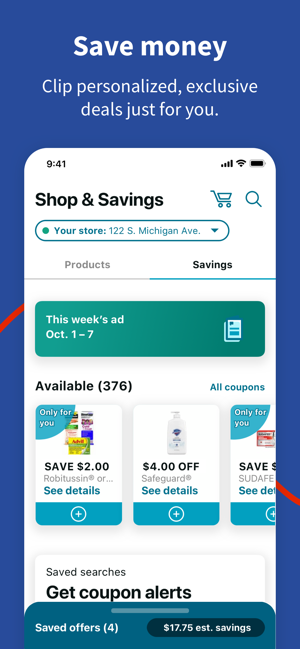A smartphone screen displays an app designed for personalized savings and exclusive deals. The app features a predominantly blue background that darkens towards the top, accented by a couple of red curved lines emerging from behind a pop-up window resembling the shape of a smartphone screen. 

At the top of the screen, the device status is visible, showing the time as 9:41, along with signal bars, Wi-Fi, and battery indicators. Below the status bar, the app title "Shop and Savings" is displayed alongside icons of a magnifying glass and a shopping cart. Beneath this, there is a location indicator, "Your Store: 122 South Michigan Avenue," accompanied by a down arrow for changing the location.

The interface features two main tabs: "Products" and "Savings," with "Savings" currently selected, indicated by teal underlined text. Just below the tabs, the app presents a floating field with a heading "This Week's Ad, October 1-7," and an icon of two pages on the right side.

The content area displays several deal items, extending off to the right, with only two and a half items fully visible. The first deal shows a "FOR YOU" badge with "Save $2 on Robitussin" and a circle icon with a plus sign on a blue background, indicating more details can be accessed. The Robitussin deal emphasizes the exclusivity of the offer. Next, there is a deal highlighting "Save $4 on Safeguard," illustrated by an image of a hand pump lotion dispenser. The following item is partly visible and appears to be an offer on Sudafed but is cut off.

At the bottom of the screen, there's a section that reads "Save searches, get coupon alerts," suggesting users can keep track of offers. The saved offers currently show an estimated savings of $17.75.